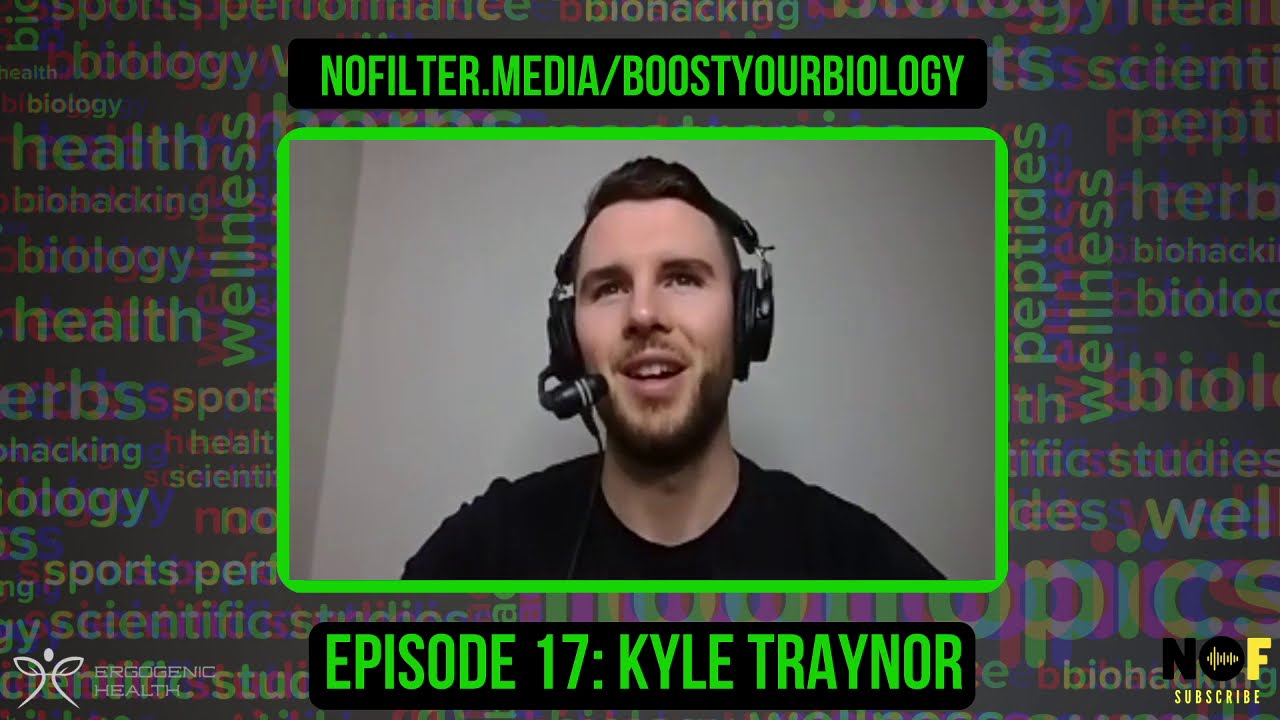This image appears to be a promotional screenshot for a podcast or informative show. At the center, there is a white man with short hair and a stubble beard, wearing a black shirt and a headset with a black microphone. He is speaking and looking slightly upward. The background features a white wall.

Framing the man's image is a bright green rectangular border. Above this border, the text "nofilter.media/boost your biology" is displayed in bright green against a black rectangular backdrop. Below the man, also in green text, it reads: "Episode 17: Kyle Traynor."

Scattered around the image are various key phrases related to the episode’s themes, including words like "wellness," "studies," "biology," and "health," appearing both vertically and horizontally. 

In the bottom corners, additional elements are present. On the bottom right, there is a bright yellow logo combining the letters "N" and "O" with vertical dashed lines resembling a voice signal, followed by an "F." To the right of this logo, the word "subscribe" appears in bright yellow text. On the bottom left, the name "Ergogenic Health" is stated alongside a unique logo depicting a human figure with leaf-like arms. 

Overall, the image features a clean modern aesthetic with predominant colors being green, black, yellow, and white, creating a vibrant and engaging visual representation for the media content being promoted.